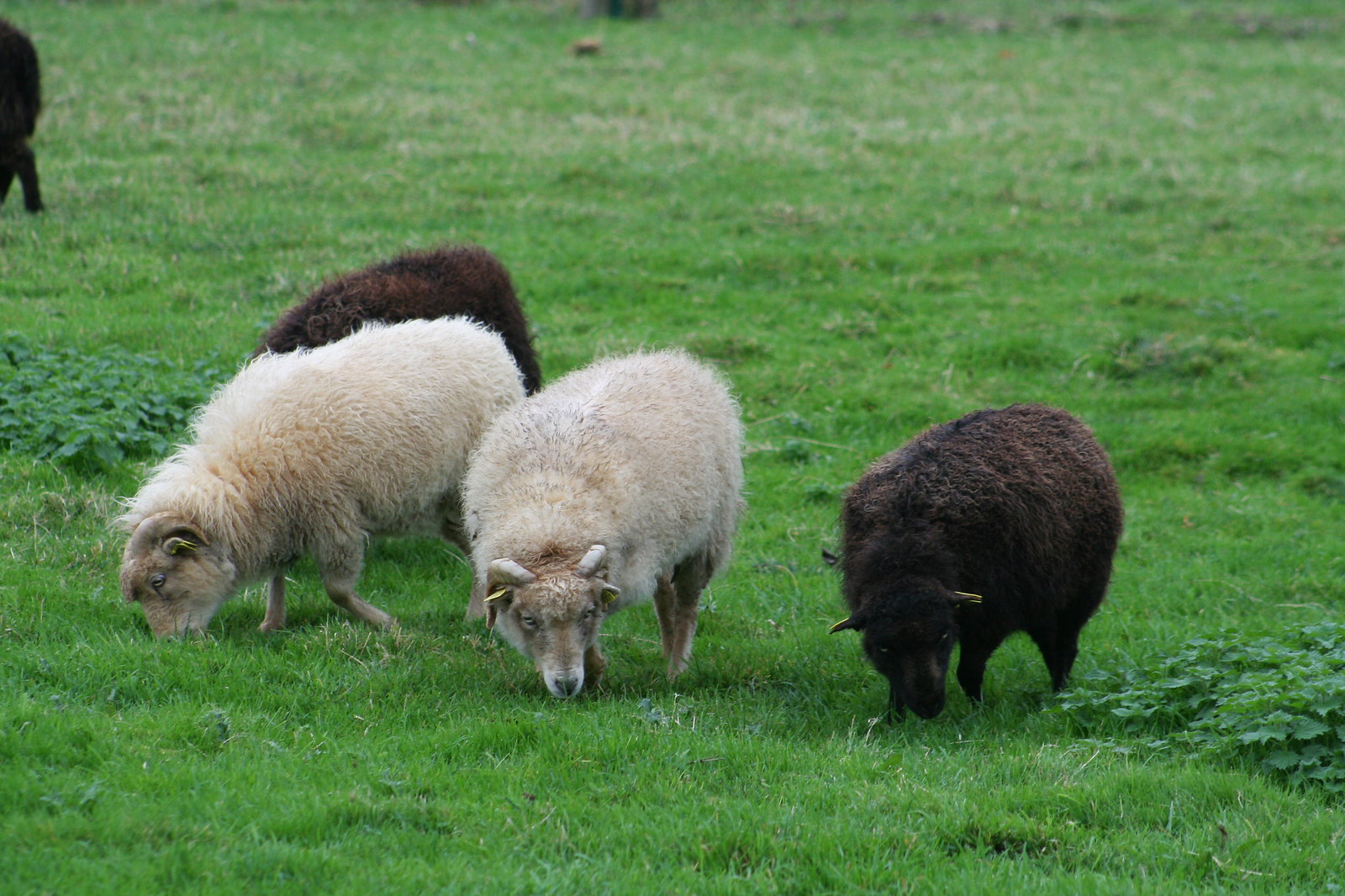In this outdoor, daytime photograph, a herd of sheep is grazing on a lush, light green grass field with some sporadic shrubbery and other greenery. Prominently featured in the mid-ground of the picture are four sheep with their heads down, munching on the grass. On the right is a black sheep with dark brown and black fur, while to its left, two beige sheep with curved horns are positioned, both also engrossed in grazing. One of these beige sheep has a noticeable ear tag. To the far left, there is a partial view of another sheep, and farther in the background, behind the beige sheep, a bit of another black sheep is visible. The scene is enveloped by the grassy field, which appears lush despite some brown patches and intermittent foliage. The ambiance suggests a possibly overcast day.